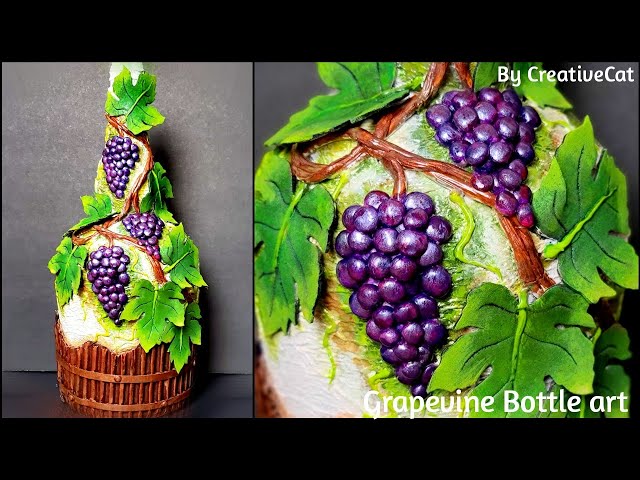The image features a detailed ceramic bottle designed as a piece of grapevine art. The base of the bottle resembles a brown wooden barrel, complete with visible lines and grooves, giving it a rustic appearance. Extending from the middle of the bottle to the top, intricate 3D designs depict green leaves and clusters of deep purple grapes, mimicking the look of a grapevine. The leaves appear to be made of fake materials, sticking out in a 3D manner, adding texture and depth to the bottle. The grape clusters, resembling small purple-painted pebbles, hang naturally from the 'branches'. The scene has a grey background and floor, giving a neutral backdrop that highlights the bottle's vibrant artistry. Additionally, there's black letterboxing at the top and bottom of the image, with text reading "buy creative cats" on the top and "grapevine bottle art" on the bottom right. The image is split into two views: a left, zoomed-out perspective showing the entire bottle and a right, close-up view that details the artistic elements and craftsmanship.